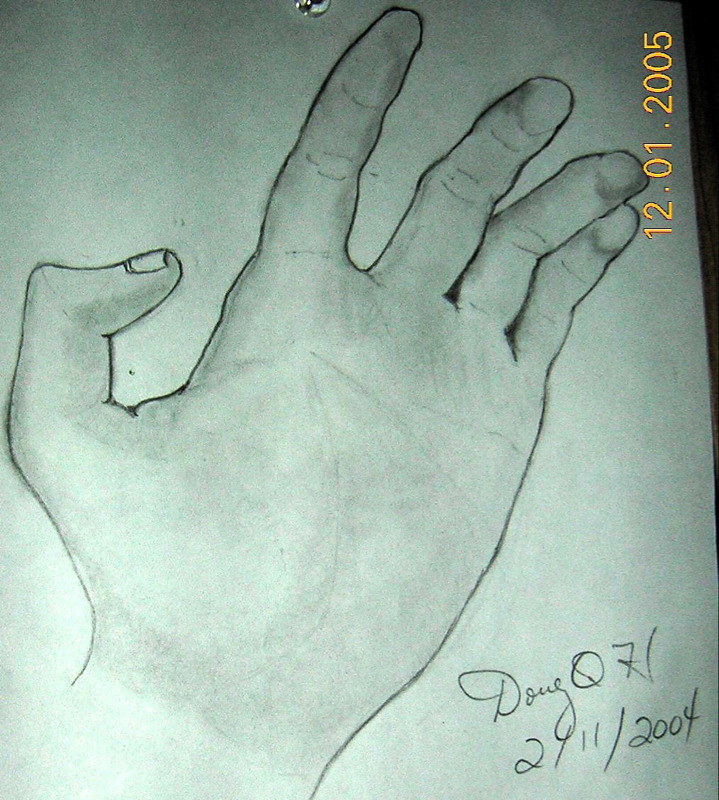The image showcases a detailed pencil sketch of a right hand on a piece of drawing paper. The hand is depicted palm up with intricate shading that accentuates the anatomy; the thumb is noticeably bent inward, while the index, middle, and ring fingers show slight bends, especially towards the knuckles, with the pinky also partially bent. The sketch features carefully drawn palm lines and shading variations, from light gray to darker tones, particularly under the thumb, between fingers, and at the edges where the fingers touch. To the right of the hand, the name "Doug" is written in cursive, followed by what appears to be an "O," a 7, and possibly a 1. The date "2/11/2004" is also inscribed below the hand. The photograph of the drawing bears a digital timestamp in orange in the top right corner, indicating it was taken on December 1st, 2005.